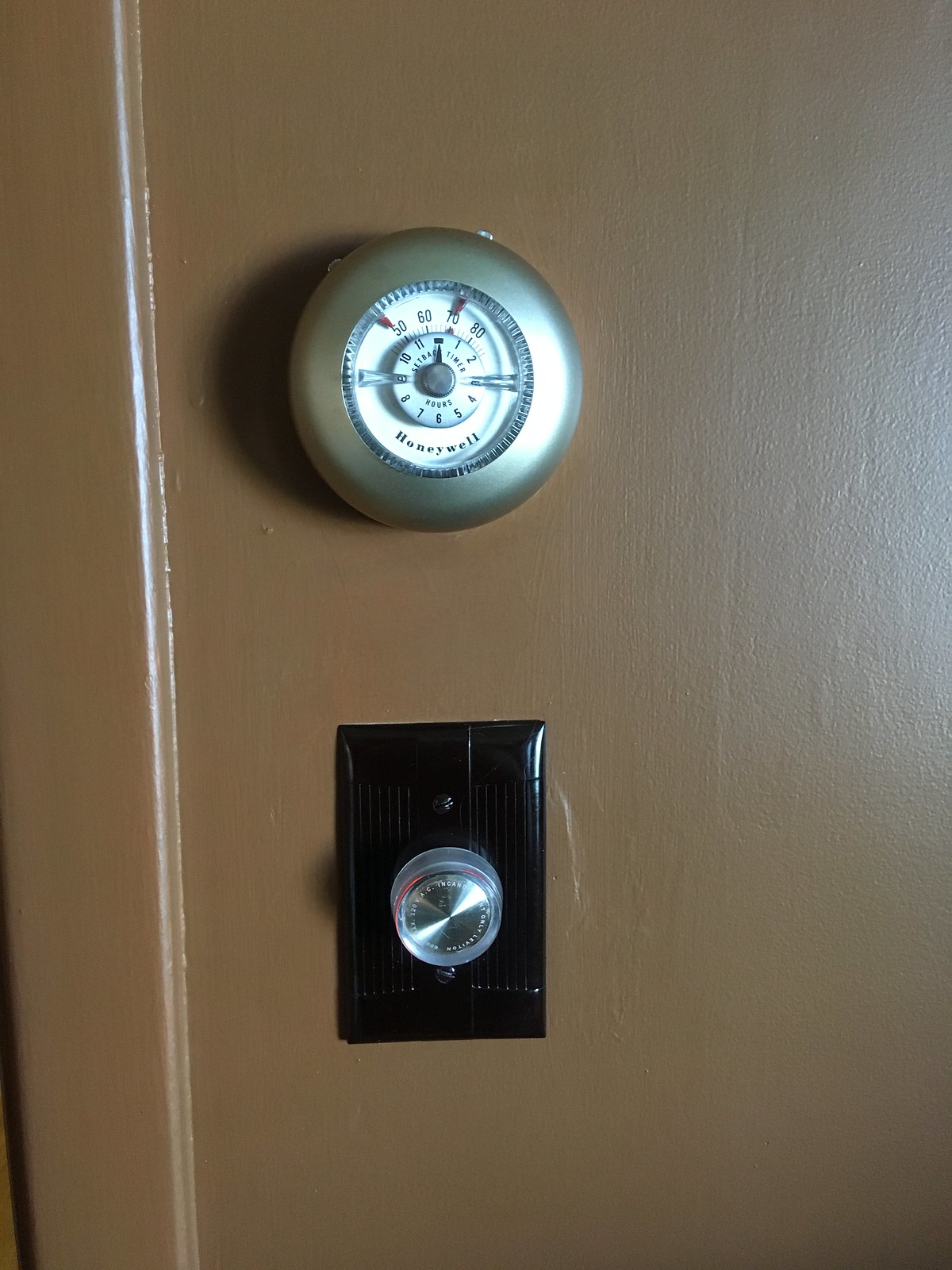A medium-brown wall features two distinct fixtures. The first is a modern, circular dimmer light switch with a black faceplate and black screws, seamlessly blending into the décor. Above it, mounted on the wall, is a vintage-style Honeywell temperature gauge. The gauge has a goldish hue and displays temperatures ranging from 50 to 80 degrees Fahrenheit, designed to resemble a classic clock face, adding a touch of retro charm to the interior.